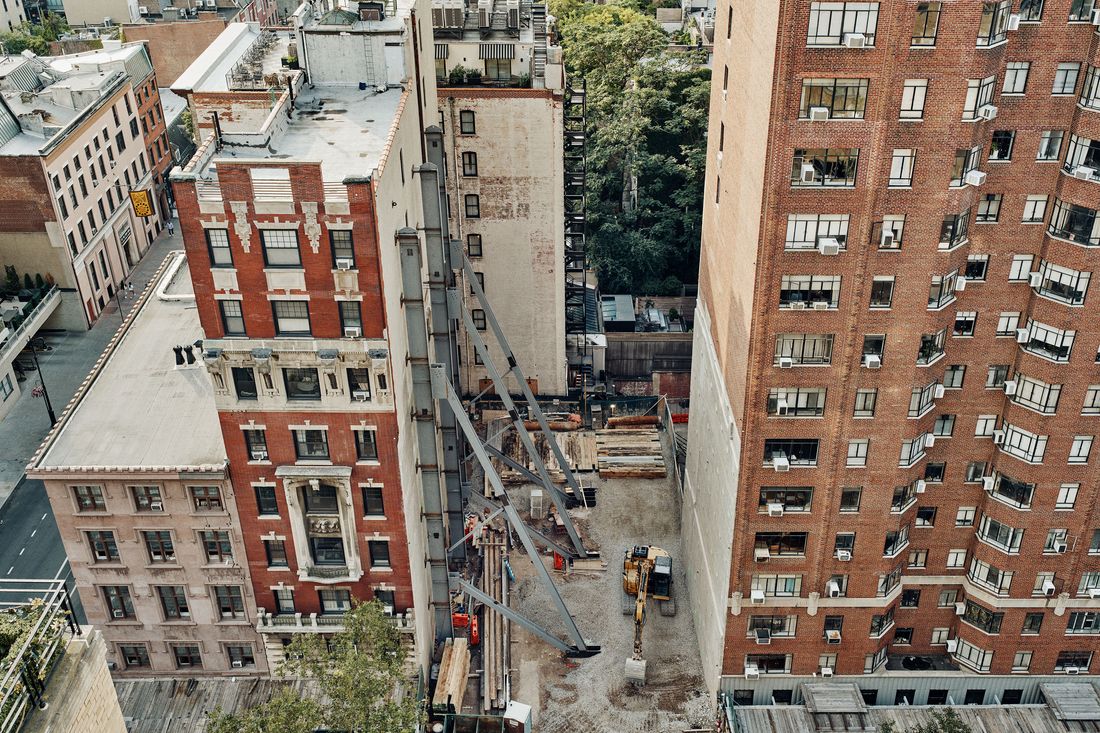A full-color photograph taken during the daytime in a bustling city captures a scene dominated by construction activities. The right side of the nearly square image is occupied by a multi-story brown brick building, featuring many closed windows and numerous window unit air conditioners but no visible people. Centrally, at ground level, heavy construction equipment, including a large digging machine, is actively working in a plot of land demarcated for future development. Scaffolding, metal beams, and wooden planks are scattered around, suggesting a significant building project in progress. Adjacent to the construction site, another smaller brown brick building stands, succeeded by a brighter red brick structure that is also under construction. This red building contrasts with a shorter, approximately four-story-high beige building nearby. The left side of the photograph reveals a street lined with additional brown brick buildings, encapsulating the urban environment amidst ongoing development.